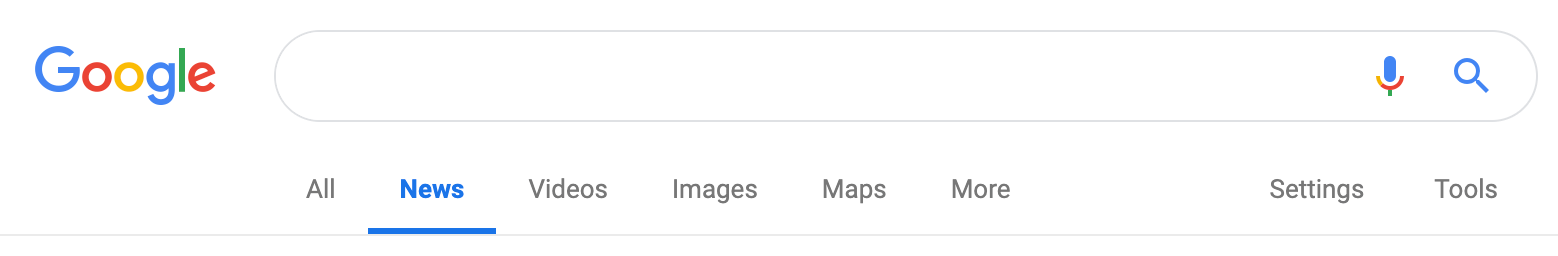The image depicts a small and detailed snippet of a Google search bar. Prominently displayed on the top left is the iconic Google logo. The logo features the word "Google" with distinctively colored letters: the capital 'G' and the lowercase 'g' in blue, the first 'o' in red, the second 'o' in yellow, the 'l' in green, and the 'e' in red.

To the right of the logo is an empty white search bar, outlined in light gray, shaped like a horizontal oval. On the far right side of this search bar, there is a detailed, colorful microphone icon. The top part of the microphone is blue, with a red and yellow curved section beneath it, followed by a vertical green line.

Adjacent to the microphone icon is a blue magnifying glass, oriented diagonally with the magnifying portion facing the top right, and the handle facing the bottom right.

Beneath the search bar, several menu options are visible in a horizontal line. From left to right, the text reads: "All" in gray, "News" in bold blue text, "Videos" in gray, "Images" in gray, "Maps" in gray, and "More" in gray. Further to the right, additional options include "Settings" in gray text, and "Tools" in gray text.

Notably, there is a prominent blue line protruding underneath the word "News," indicating the currently selected category. The other menu options are underlined with a thin, light gray line.